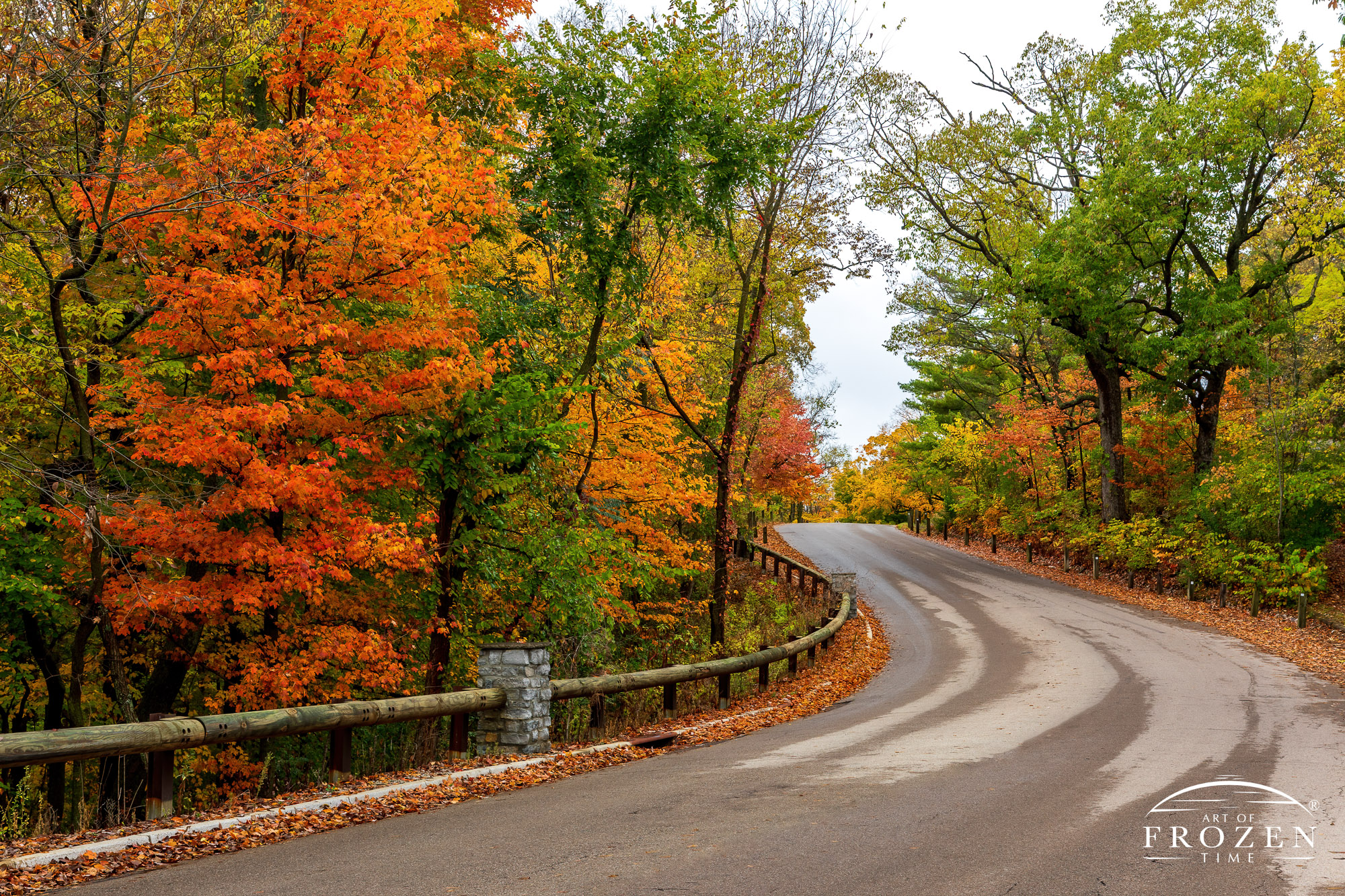An outdoor photograph captures a picturesque country road during early autumn, winding gracefully from the bottom left, curving to the right, and then bending back towards the left into the distance. The paved roadway is slightly wet in places with a few dry patches, particularly on the right side. The left edge of the road is bordered by a wooden split rail fence connected by stone pillars, seemingly providing safety along what appears to be a slight drop. Both sides of the road are adorned with clusters of deciduous trees in various stages of their fall transformation: bright red, yellow, orange, and green leaves create a vibrant tapestry in the midground and background. Notably, a brilliant orange-leafed maple stands prominently on the left edge, further surrounded by dense groves of trees in varying autumn hues. The ground is scattered with fallen leaves, reflecting the season. The sky above is overcast, casting a diffuse white light over the scene. In the bottom right corner, there's a logo reading "Art of Frozen Time," with a registered symbol, lending a touch of artistic branding to this serene landscape.